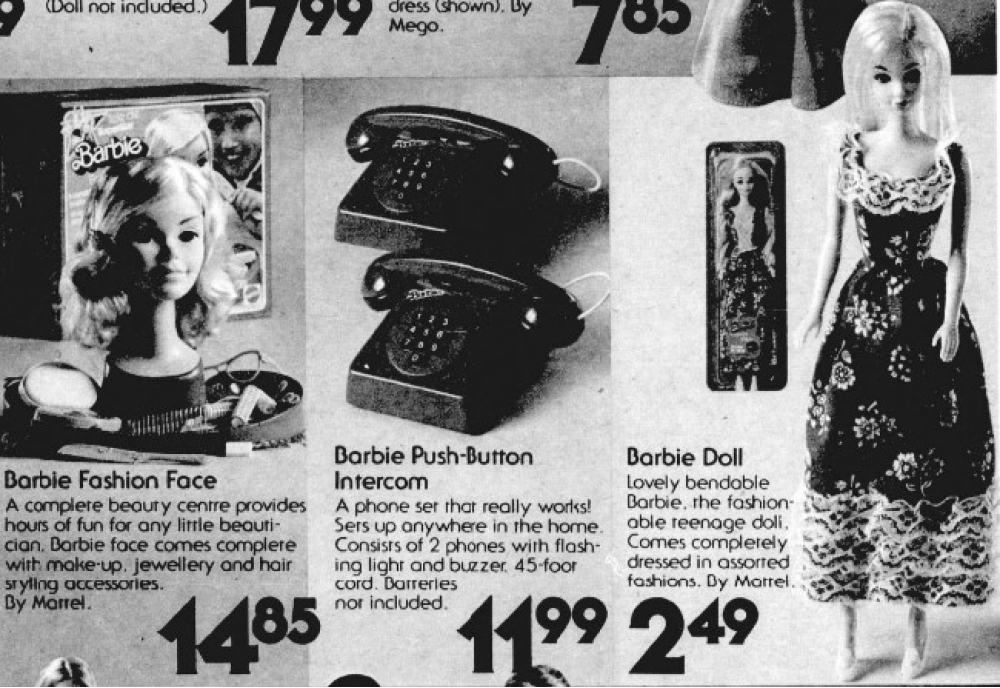This black and white newspaper advertisement showcases a variety of Barbie products from Mattel, highlighting their affordability and features. 

On the far left, there's the "Barbie Fashion Face," a comprehensive beauty center designed to provide hours of fun for aspiring young beauticians. The set includes makeup, jewelry, and hairstyling accessories, all for $14.85. The image prominently features a large, human-sized Barbie head surrounded by various beauty accessories.

In the center column, the ad features the "Barbie Push Button Intercom," a functional phone set resembling old rotary phones but with a push-button keypad. This set, priced at $11.99, includes two phones with flashing lights, buzzers, and a 45-foot cord, although batteries are not included.

The far right column showcases the iconic "Barbie Doll," described as a lovely, bendable, fashionable teenage doll. This Barbie comes fully dressed in assorted fashions and is available for just $2.49. The visual displays the doll both outside and inside its box, emphasizing its appeal and affordability.

Overall, the ad captures the nostalgic charm and value of classic Barbie products from a bygone era.